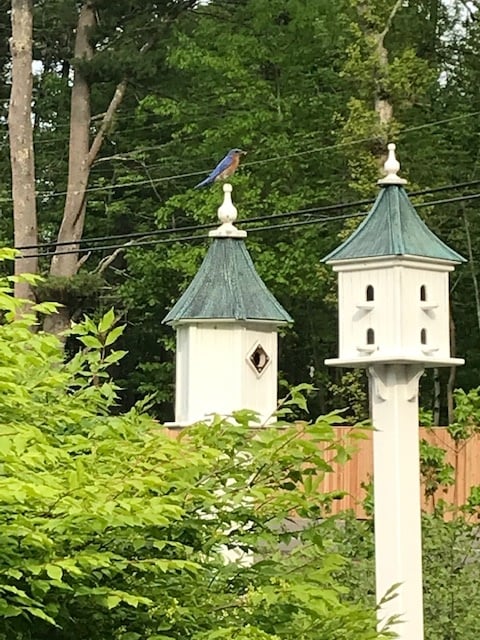This outdoor photograph features two birdhouses prominently in a lush, tree-lined setting with a wooden brown fence at the bottom. The birdhouse in the foreground, positioned slightly to the right of the center, has a distinctive green, pointed roof with a yellow steeple on top, upon which rests a bird with vivid blue feathers and a red breast. This birdhouse is yellowish and square-shaped, featuring four little entrances. To the left of this, partially obscured by green leaves, is another birdhouse with a similar green pointed roof but without the perches. Both birdhouses are mounted on white posts, which are partly visible and blend in with the surrounding greenery. In the background, the scene is filled with trees bearing lush green leaves, and electric lines stretch from left to right. At the bottom left, a large leafy green shrub adds to the verdant atmosphere.